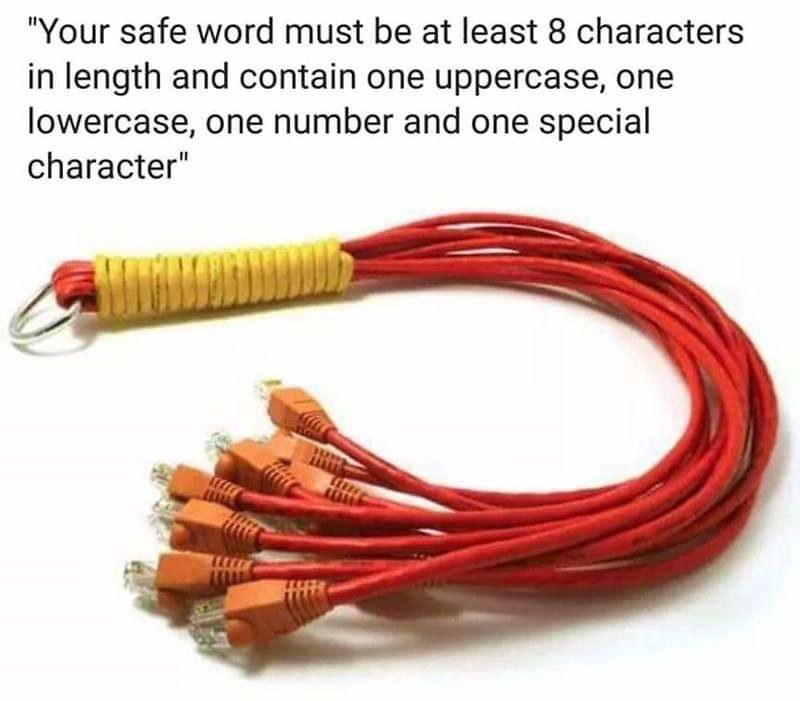The image features a white background with black text at the top, set in quotation marks, which reads: "Your safe word must be at least 8 characters in length and contain one uppercase, one lowercase, one number, and one special character." Below the text is an edited photograph of a bundle of red Ethernet cables, each with orange housing around the connectors. The cables are tied together at the base with a yellow zip tie. Extending past the point where the cables are tied is a small, bright silvery metal hook. The photograph is simple and straightforward, emphasizing the vivid colors of the cables and the clear, structured message above.